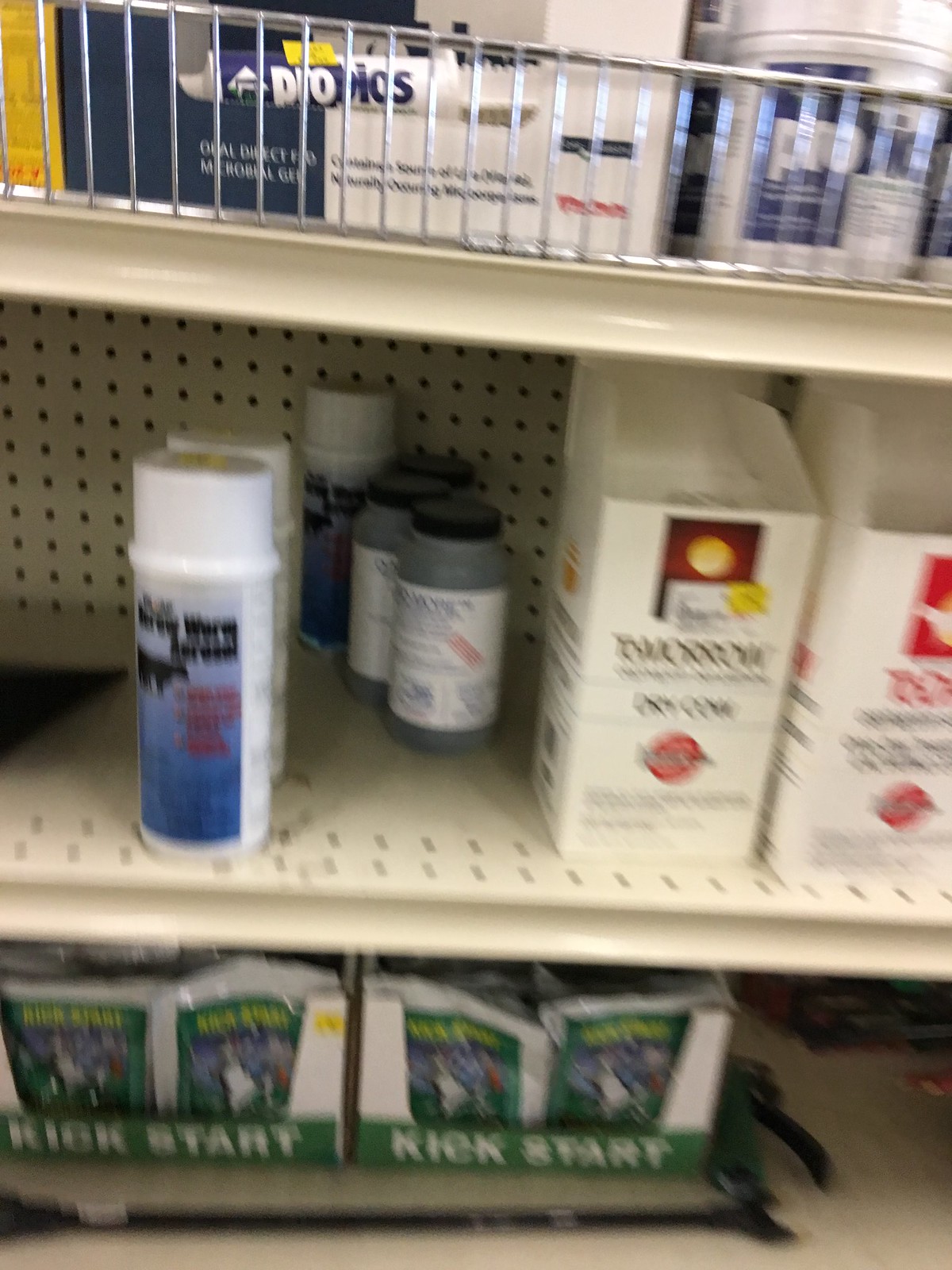This photograph captures the inside of a drugstore, focusing on the myriad of products displayed on its shelves. 

### Bottom Shelf:
The bottom shelf is slightly out of focus, showcasing products branded as "Kickstart". The notable "Kickstart" packets feature a visually striking design, with the product name "Kickstart" appearing in white against a green background. Each packet has a white border with green and blue hues and an ambiguous white graphic in the center of the logo.

### Middle Shelf:
On the middle shelf, the left side holds spray cans adorned with blue logos. Next to them are gray bottles with white labels, though the specific branding or product type is unclear. Further to the right, there are two predominantly white boxes labeled with something related to "dry", suggesting a possible skincare product. These boxes also feature a red circle logo near the bottom and a red square near the top of their design.

### Top Shelf:
The top shelf is equipped with a metal basket lining its edge. Within this basket, there is a box labeled "oral direct something microbial gel", characterized by a blue and white color scheme. The exact text is partially obscured by the metal, but it appears to include the words "probe" and "bios". Additionally, there is a matching white and blue tub to the right of this box.

The shelves themselves are cream-colored, featuring typical perforations seen in retail displays. The detailed arrangement of various skincare and health products reflects the organized yet dense layout of a typical drugstore aisle.